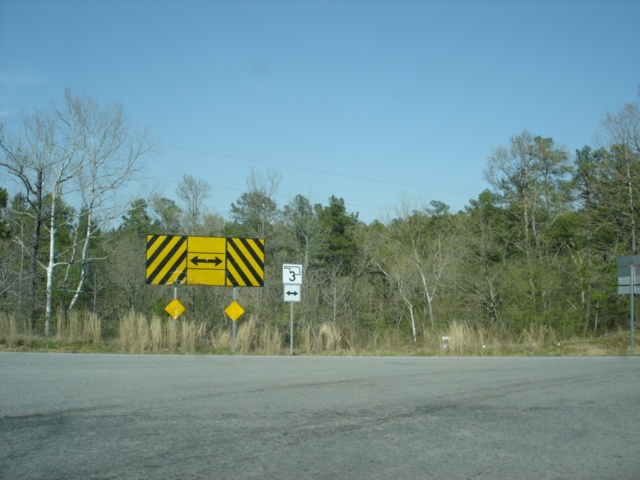A photograph of a country road, showcasing a prominent road sign on the left side. The main sign is large and rectangular, framed on either side by three smaller squares with diagonal black and yellow stripes. Centrally placed on the sign is a yellow panel with a black arrow indicating a sharp turn, flanked by two additional arrows. Below this sign, it's supported by a pair of steel beams, each adorned with a yellow triangular sign, likely reflective for visibility at night. Adjacent to these signs is a small white sign with the numeral "3" and another white sign beneath it displaying a black arrow with arrows at both ends. The background reveals a dense row of trees, including birch and pine, suggesting a winter setting due to the absence of leaves. The sky is a clear, vibrant blue, adding to the crisp atmosphere of the scene.